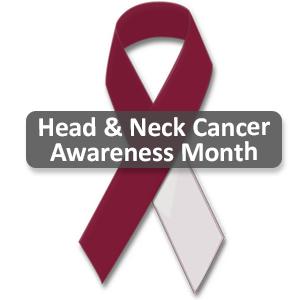The image features a folded awareness ribbon, symbolizing Head and Neck Cancer Awareness Month. The ribbon loops at the top with one side in burgundy and the other in white, specifically with the right tail being white. Overlaying the ribbon is a semi-transparent, rounded gray rectangle, centrally placed and containing the text "Head & Neck Cancer Awareness Month" in white, with each word capitalized and using an ampersand. The entire composition rests on a white background, emphasizing a minimalist yet impactful design meant to catch the public's attention and spread awareness about this specific type of cancer.